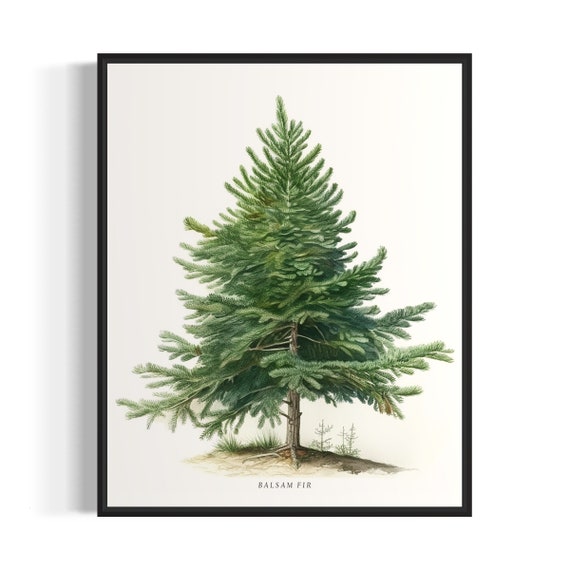This is a close-up photo of a framed colored pencil drawing of a very full and lush balsam fir tree. The tree's pine needle branches jut out from all angles, revealing a hint of a skinny, light brown trunk with darker striations. The base of the tree has visible roots intertwining with the earthy ground, where you can also see saplings and a segment of green, spiky grass and weeds. The drawing, set against an off-white canvas, is encased in a thin black frame. The detailed illustration shows the tree gradually tapering at the top, with varying shades of green depicting its fluffy, bountiful foliage. At the bottom of the drawing, the label "BALSAM FIR" is clearly inscribed in capital letters. The color scheme of the artwork includes green for the tree, grass, and saplings, brown for the trunk and branches, and black and white for the background and frame.